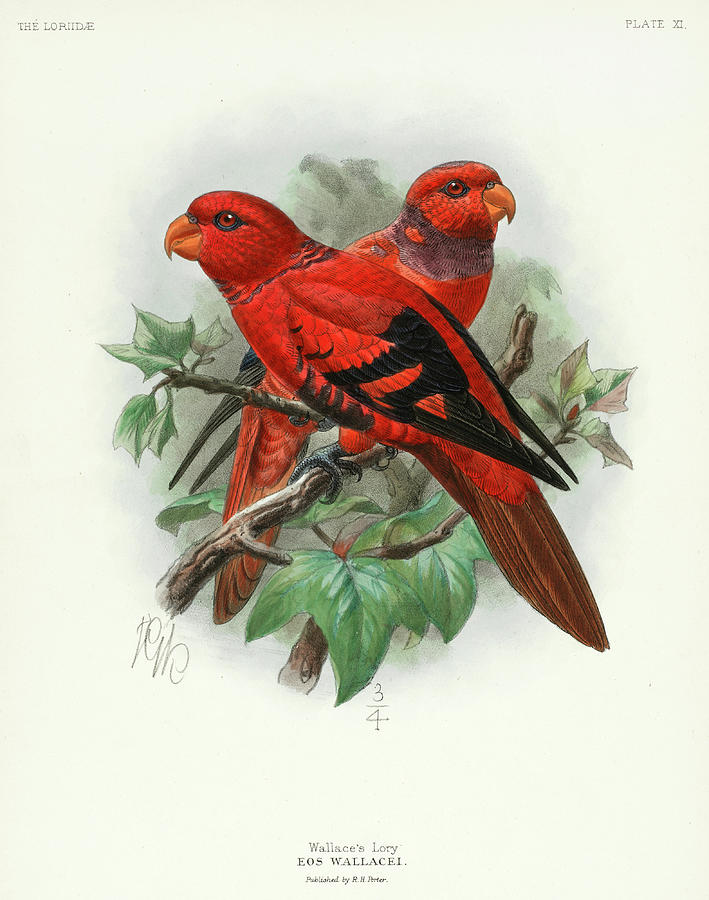This illustration, titled "Wallace's Lory, E. H. Wallace C., published by R. H. Peter," features two vividly drawn red birds positioned centrally on a crisp white background. The birds, reminiscent of lories or parakeets, are intricately detailed with bright red plumage, highlighted by orange beaks and dark red eyes. Their feathers exhibit subtle yet distinct touches of black edging and brown tail tips, while the upper neck areas showcase fine lines and purple patches. Set amid delicate green leaves and branches, the birds are portrayed standing one behind the other, facing opposite directions, with the left bird looking left and the right bird looking right, possibly indicating a mated pair. The top left corner of the illustration reads "The Lory Day," and the top right is marked "Plate 11." The detailed leaves and branches blur into a gray background, ensuring that the brilliantly colored birds are the focal point of this meticulous artwork.